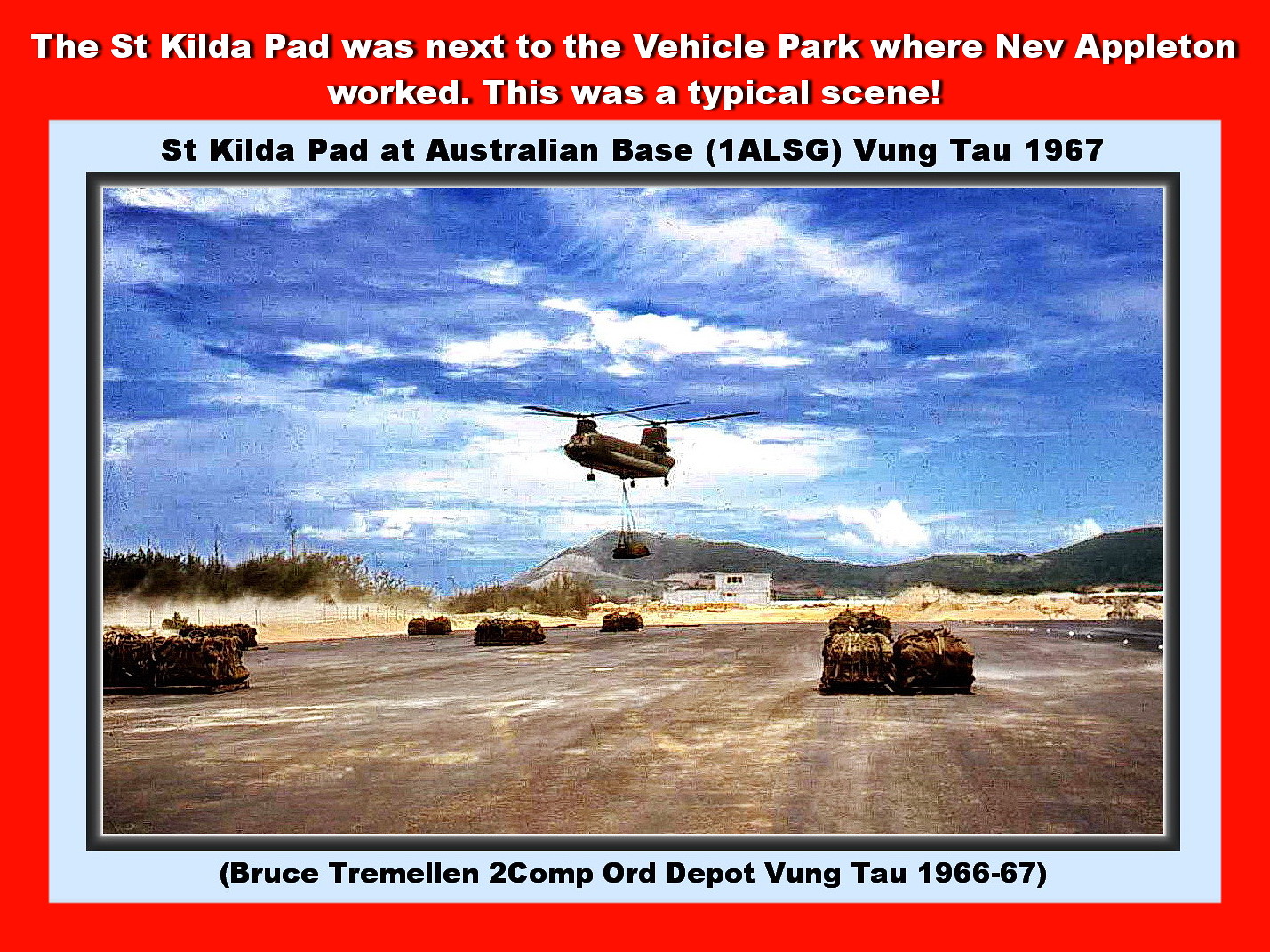A vintage postcard with a red border encapsulates an old color photograph. The red border frames the image and bears white text at the top reading, “The St. Kilda pad was next to the vehicle park where Neve Appleton worked. This was a typical scene.” Within this red border is a blue border, and inscribed on the top of this blue border in black text is: “St. Kilda pad at Australian base, (K-I-L-L-S-G), Vung Tau, 1967.” At the bottom of the blue border is further text: “Bruce Tremelin, 2 Comp, Ord Depot, Vung Tau, 1966-67.”

The photo within these borders captures a military scene with a transport helicopter hovering close to the ground, carrying cargo suspended beneath it. Below, scattered on what appears to be an airfield or runway are about five tanks. In the background, rugged mountains rise under a dramatic sky that appears stormy and threatening. The entire image portrays a significant moment from the Australian base at Vung Tau during the Vietnam War era.